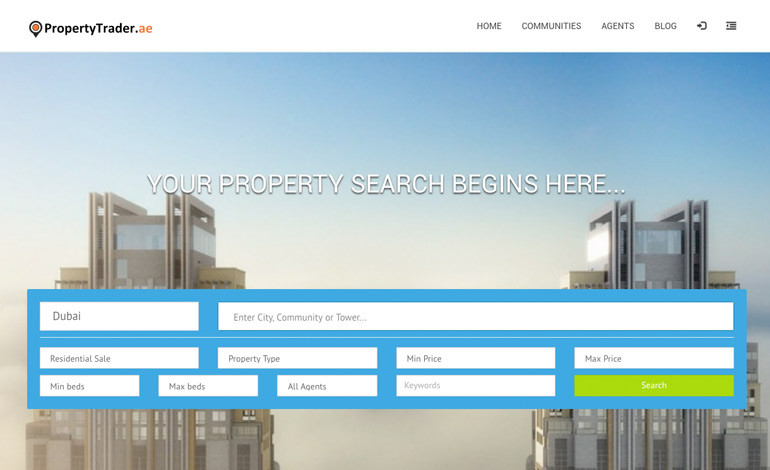This image depicts the home page of PropertyTrader.ae, showcasing an organized layout designed for property search. In the upper left corner, there is a pin symbol encased in an orange circle, adjacent to the site's name "Property Trader" in bold black text with "AE" highlighted in orange. 

At the top of the page, a navigation bar features columns labeled Home, Communities, Agents, Blog, along with several symbols for additional functionalities. Dominating the visual is an impressive photograph of two modern skyscrapers, adorned with sleek metal railings and vast arrays of windows encircling both towers. The backdrop presents a vivid blue sky generously dotted with clouds, adding depth and liveliness to the scene.

Positioned across the lower section of the skyscraper image is a striking turquoise banner stretching almost the full width. Prominently placed above the banner is the inviting phrase, "Your Property Search Begins Here." Below this heading, the turquoise banner is segmented into three distinct rows of user-friendly search bars.

- The first row presents a dropdown menu initialized to "Dubai," allowing for location-specific searches.
- The second row offers fields labeled "Enter city, community, or tower," alongside options for "Residential Sale," "Property Type," "Min Price," and "Max Price."
- The third row includes fields for "Min Beds," "Max Beds," "All Agents," and "Keywords," culminating in an easily noticeable green "Search" button.

This detailed and intuitive layout is clearly designed to facilitate a seamless and efficient property search experience for users.